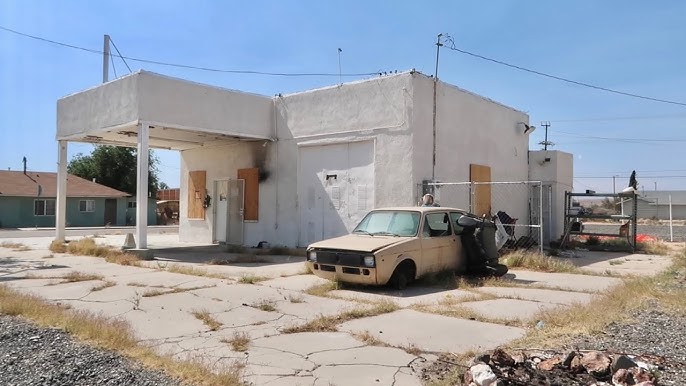The photograph portrays an abandoned, old-fashioned building that appears to have once been a car garage. The structure is primarily white concrete with boarded-up windows and a garage door, supported by two pillars holding up an overhang. The building shows signs of neglect, including broken and cracked concrete around it with grass and dead weeds sprouting through the gaps. The ground beneath features both gravel and large stones. The building has smoke damage near one window, possibly indicating a past fire, and a door that hangs off its hinges. 

In front of the structure, there is a deteriorating car, a mix of eggshell white, tan, and yellow with a black front grill, missing pieces, and no tires, suggesting it has been abandoned for quite some time. The vehicle is positioned diagonally to the building, with an object protruding from its right side.

To the side, remnants of a dark gray gate and a partially standing chain-link fence can be seen. In the distance, there is a dark green house with a tree behind it, as well as a small blue house. The scene is set under a clear blue sky, which contrasts with the desolate and forgotten atmosphere of the foreground.